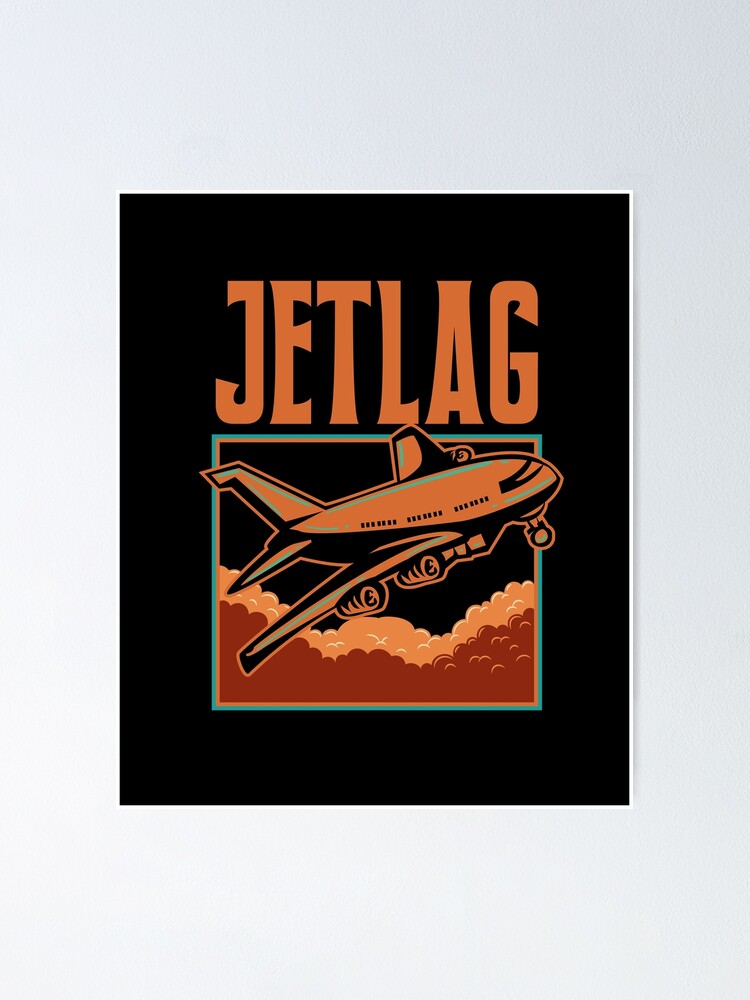The image appears to be a highly stylized and detailed graphical illustration, possibly designed for the front cover of a magazine, album, or artwork related to an airline theme. The central piece of the graphic sits on a light gray, almost white background, and is framed by a thin white outline with a subtle drop shadow effect. 

In the focal point of the image, there is a black rectangular graphic with bold, eye-catching orange text in large, capital letters reading "JETLAG" at the top. Below this header, the design features a square with a dual border—an outer aqua green and an inner orange. Inside this bordered square, a vector-style illustration of a large airplane, resembling a jumbo jet, is depicted taking off at an angle. The airplane is primarily tan and black with aqua green highlights that accentuate its wings and body.

This jet appears to be ascending above a layer of fluffy clouds, which exhibit a color gradient from white and tan to orange, enhancing the sense of depth and movement. The overall composition combines modern digital art elements with vivid colors and clean lines, making it a striking and visually captivating image.